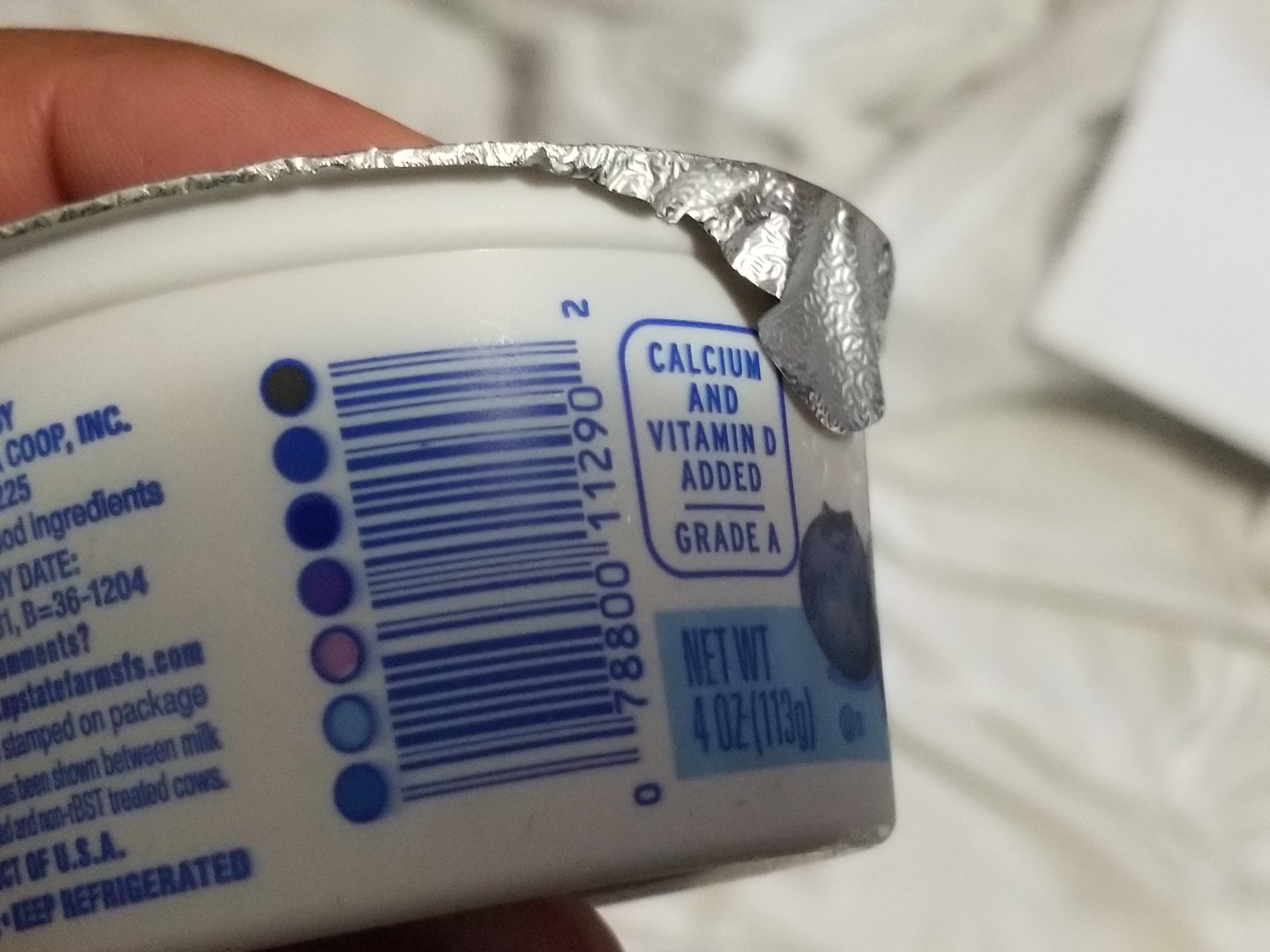The image is a close-up photograph of a single-serve yogurt container. The container has a white, pot-like shape with a thin, silver foil lid. A hand is holding the yogurt up towards the camera, making it the focal point of the image. In the background, a white fabric sheet softly diffuses the light, eliminating distractions and drawing attention to the yogurt container. The container's label is prominently visible and features blue text. Notably, there is a large barcode on the label, along with descriptive text indicating that the yogurt contains added calcium and vitamin D and is classified as Grade A. The net weight of the yogurt is 4.40 ounces, equivalent to 113 grams. Although the label includes a list of ingredients and additional information about the product, these details are mostly cropped out of the image.